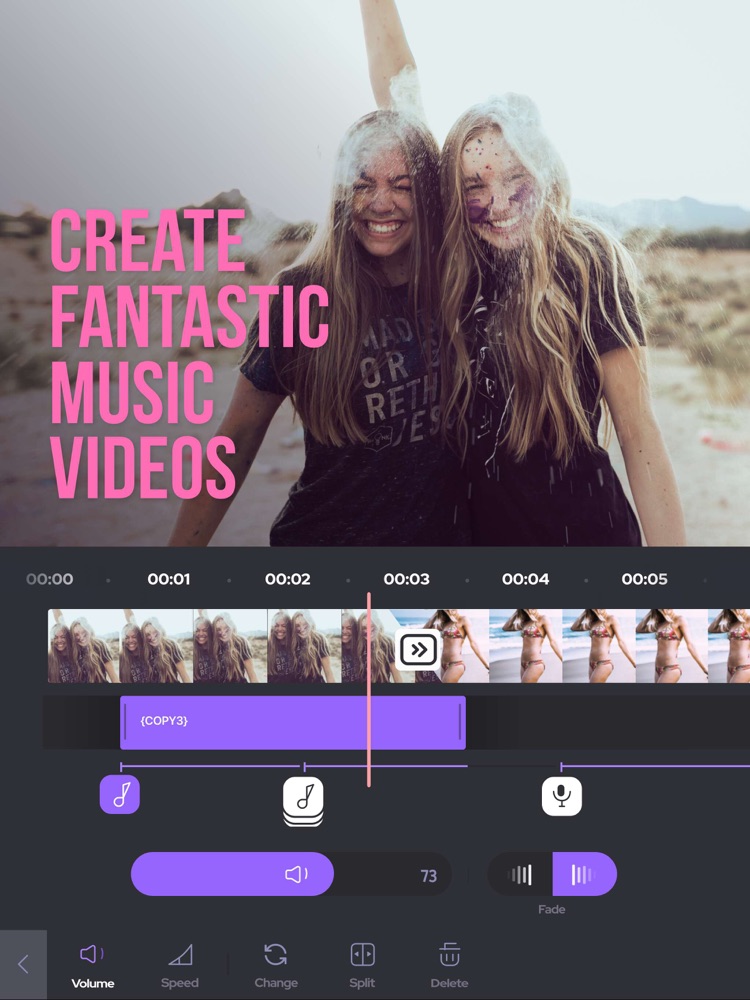This is a screenshot from a simplified video editing application, likely a mobile app. The interface features a row of editing options at the bottom, each represented by an icon. These icons include "Volume" (selected and highlighted in white), "Speed," "Change," "Split," and "Delete" (all in gray). Above this row, there are additional icons in a purple hue. A gray background with a left-pointing purple arrow can also be seen on this level.

In the middle section of the screenshot, there's a dark interface with purple highlights detailing the editing tools. This area displays options such as "Copy," presumably useful for duplicating content. There are also still images or frames from the video being edited, accompanied by numerical markers to denote specific frames or seconds in the timeline.

At the top of the interface, there's a photograph of two women with long hair, both smiling. One woman has her arm raised above her head. This scene appears to be in a desert-like environment.

On the left side of the interface, a vertical menu in pink reads "Create" at the top, followed by "Fantastic," "Music," and "Videos." The overall look of the application is dark with significant vignette effects, indicating a user-friendly, visually appealing design that seems to be aimed at basic video editing tasks rather than advanced features like those found in Adobe Premiere.